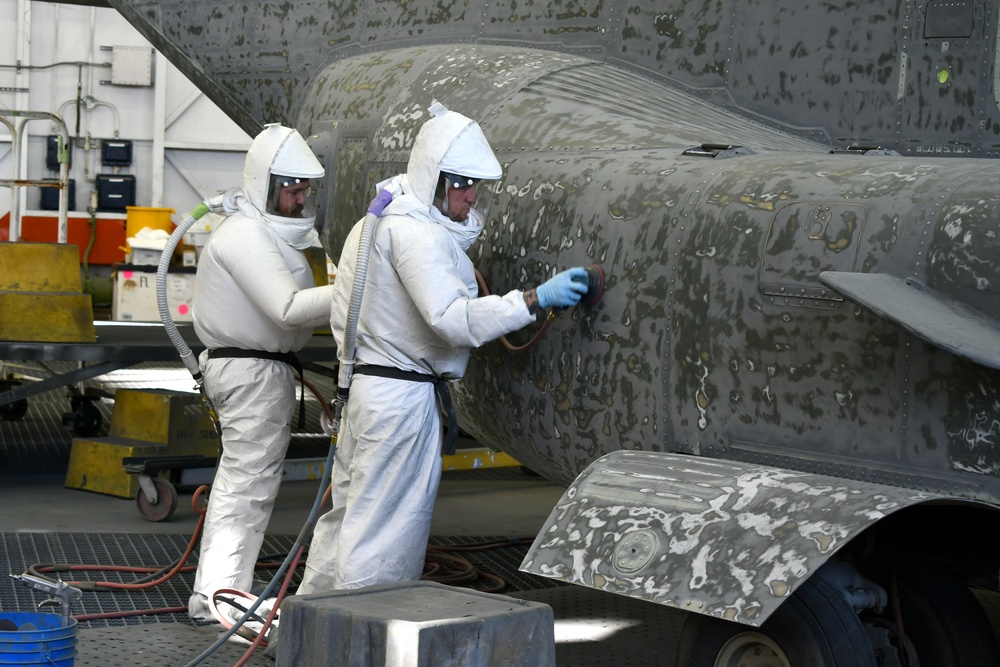In a large warehouse-like setting, two men dressed in white hazmat suits with clear visors and blue gloves are meticulously cleaning the stripped-down surface of a dark greenish, military-style aircraft. The plane, which has been mostly sanded bare of its original paint, is being prepared for what appears to be a repainting process. The men are using hand tools connected to packs on their backs, which might be part of their cleaning apparatus. Around them, the spacious interior is filled with various industrial items, including boxes, hoses, and a blue bucket in the far left corner, all contributing to the busy, industrious atmosphere where this intricate restoration work is being done.